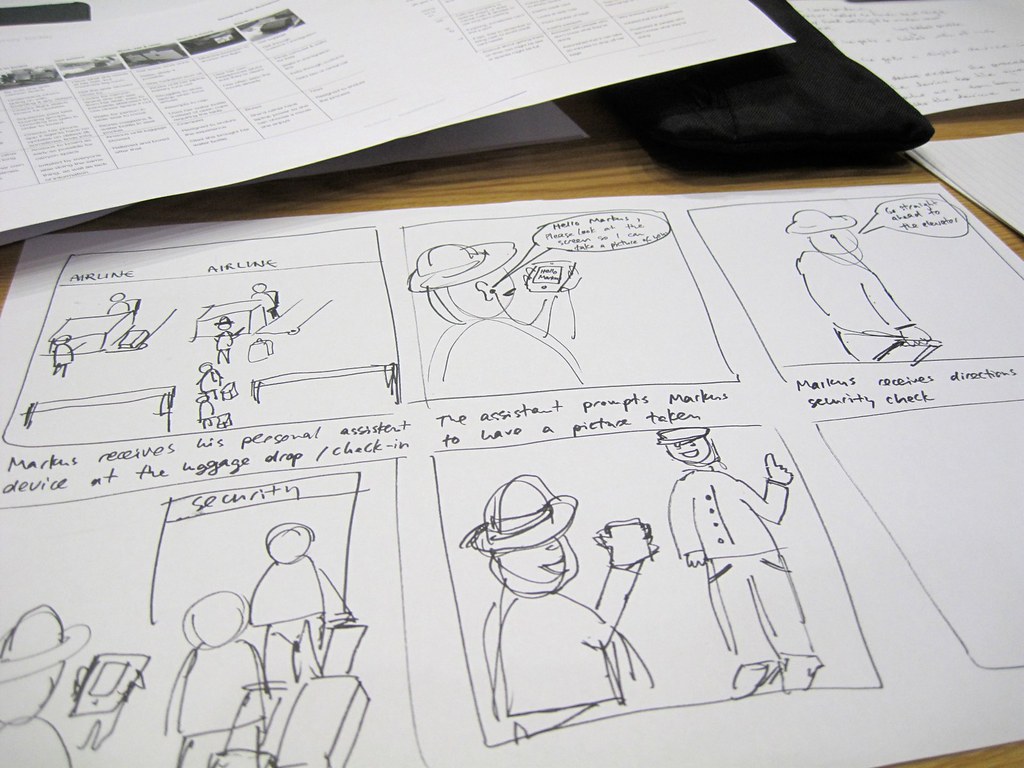The image is a color photograph of a horizontally positioned piece of white paper covered with cartoon-like sketches, similar to comic book panes. The paper, resting on a wooden table, features six rectangular boxes, arranged in two rows of three. Only five of the boxes contain sketches, each adorned with simple, hand-drawn figures and accompanying text. 

In the top left box, the text "Airline Airline" appears above a sketch of people in line at an airport, interacting with airline assistants. Below this, the text reads "Marcus receives his personal assistant device at the luggage drop/check-in." The second box depicts Marcus looking at the device, with a caption explaining that the assistant prompts him to have a picture taken. The third box is not clearly readable from the photograph. 

The bottom left box shows a security sign and Marcus, holding his device, going through a security line. The final sketch presents an official or police officer smiling at Marcus, who is still holding the device. Additionally, in the top right corner of the image, partially visible photographs with text beneath them lean against what appears to be a black pouch. This detailed storyboard or cartoon sequence likely illustrates Marcus's journey through airport procedures with the aid of a personal assistant device.